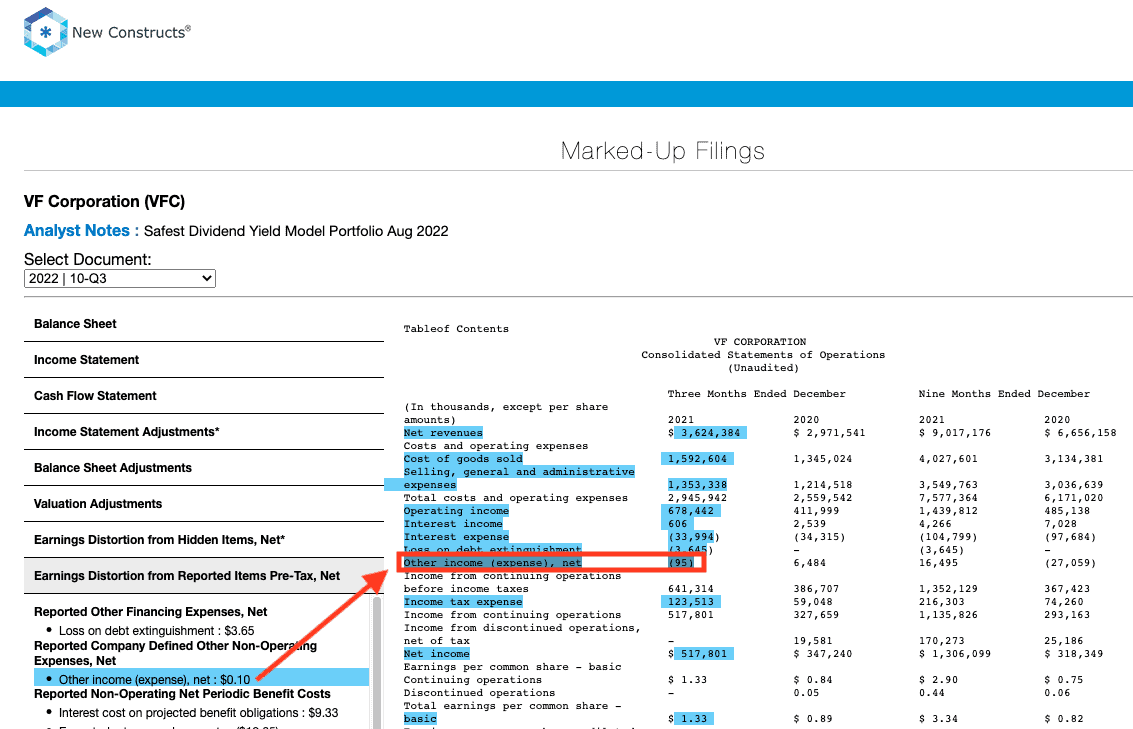The image is a detailed screenshot of a website called "New Constructs." The logo prominently featured on the site is a unique 6-sided shape resembling a snowflake at its core. The title of the page is "Marked Up Filings, BF Corporation (BFC), Analyst Notes - Safest Dividend Yield at Model Portfolio, August 2022." Below the title, there is a drop-down menu allowing the user to select the desired quarter for detailed financial information. 

The main content includes a comprehensive table outlining various financial metrics such as Net Revenue, Cost and Operating Expenses, Cost of Goods Sold, Selling General and Administrative Expenses, Operating Income, and Interest Income. There is a specific emphasis on a particular line item titled "Other Income Expenses Net" from the year 2021, highlighted by a red arrow and a red rectangle. This line item shows an amount enclosed in brackets: (95), though the exact significance is unclear. Overall, the markup provides an in-depth look at the financial details and performance indicators of BF Corporation.